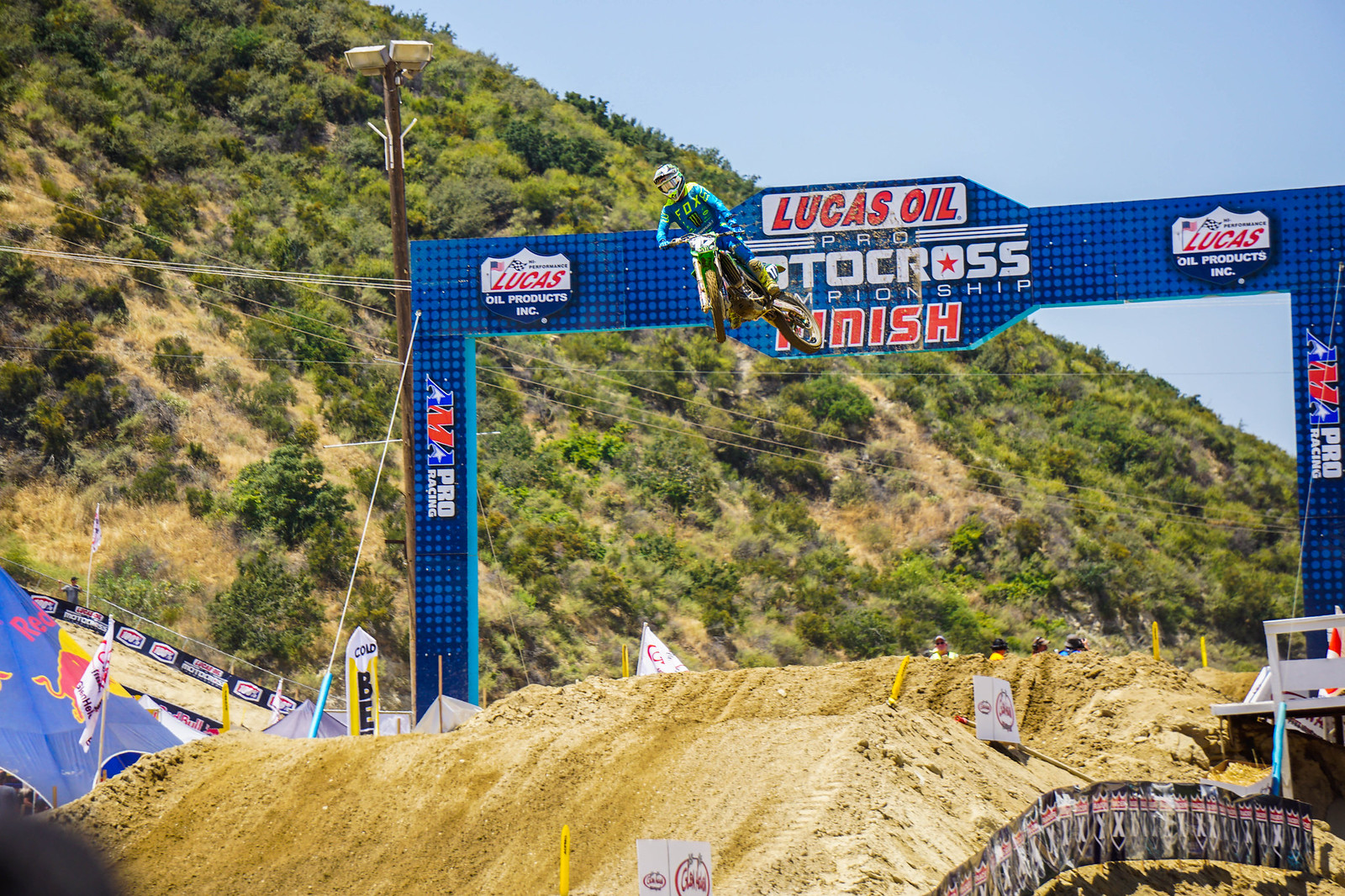This outdoor photograph captures a thrilling moment at the Lucas Oil Pro Motocross Championship. A motocross rider, adorned in a teal and yellow Fox-sponsored outfit, soars through the air after launching off a sizable dirt jump on the track. The rider’s bike, featuring yellow fenders, zips toward the camera against a backdrop of a lush, green mountainside under a light blue sky. Dominating the scene behind the airborne rider is a large, blue archway structure emblazoned with "Lucas Oil Pro Motocross Championship Finish" along with the AMA Pro Racing and Lucas Oil Products logos. Below, the dirt track is lined with several bunny hop hills and yellow markers. Also visible are some heads of spectators or riders peeking over a dirt hill in the background, adding to the dynamic atmosphere of the race. The attention to vibrant colors and brand logos, paired with the natural scenery and structural details, encapsulates the intensity and setting of this motocross event.